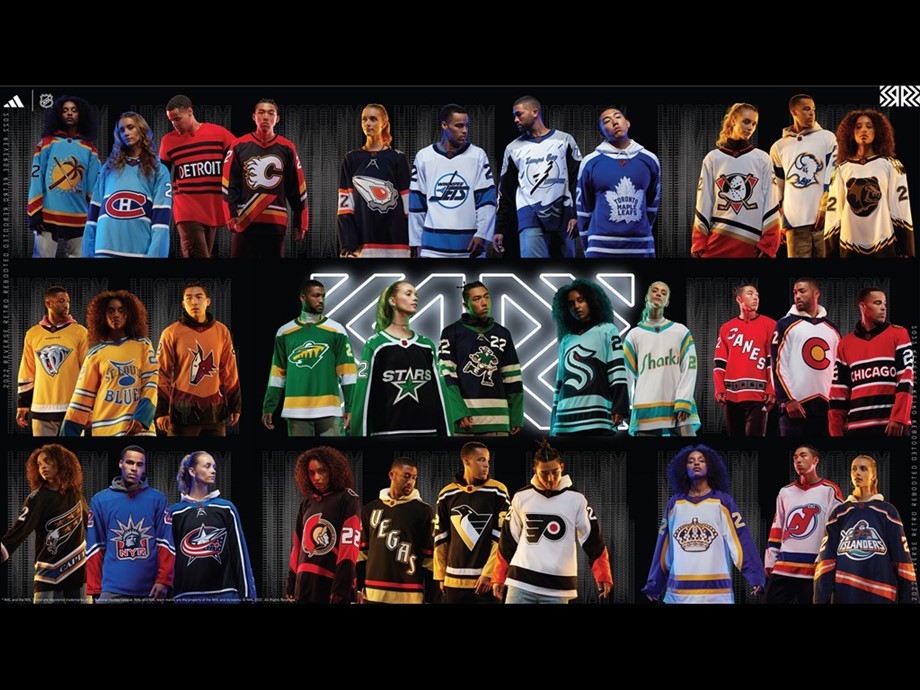This website image showcases a diverse collection of nine Adidas sports jerseys, each representing different hockey teams. The Adidas logo is prominently displayed in the upper left corner of each jersey. The models showcasing these jerseys include a diverse group: one Asian model, several Hispanic models, and multiple African-American male and female models. Each jersey is worn by athletes who exemplify the brand's inclusivity and global appeal. Despite some jerseys having designs reminiscent of football teams, they are all confirmed to be hockey jerseys.